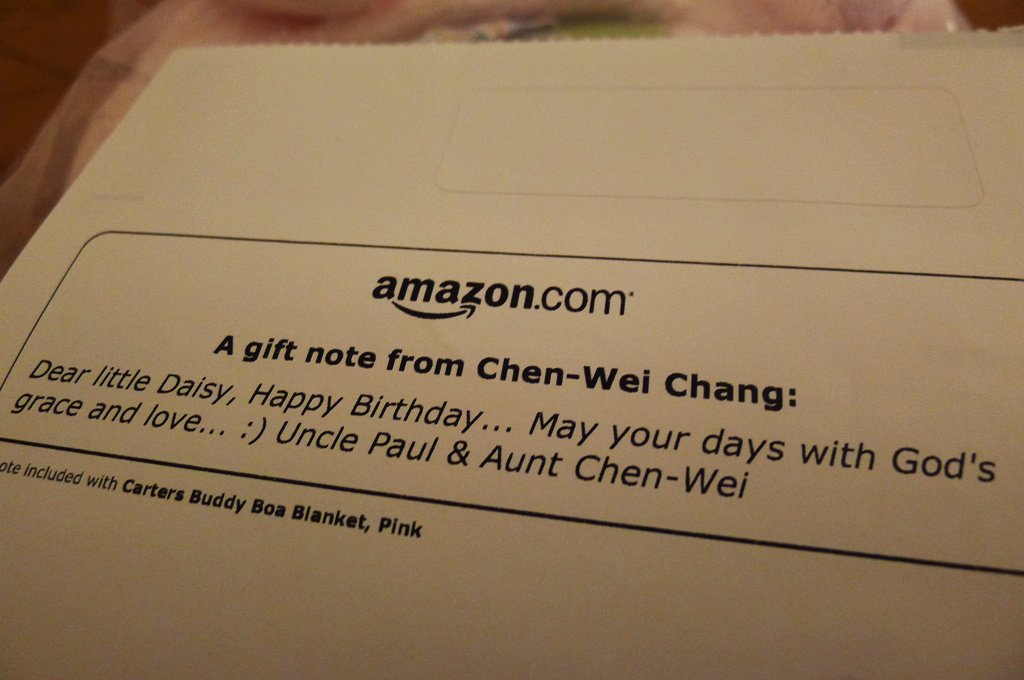This close-up photograph captures a shipping label from Amazon.com featuring a heartfelt gift note. The white piece of paper is slightly frayed at the top, as if torn from a perforated edge. At the top of the label is a blank white rectangle with a black border, followed by another black-bordered rectangle with curved corners. The top of the label prominently displays "amazon.com" in black, accompanied by the iconic arrow from "A" to "Z." Below this, in bold dark ink, it reads "A gift note from Chen Wei Chang," followed by the message: "Dear little Daisy, happy birthday. May your days be filled with God's grace and love :) Uncle Paul and Aunt Chen Wei." Toward the bottom, it notes, "Included with Carter's Buddy Boa Blanket, Pink." Subtly visible beneath the label is the pink blanket, indicating that it accompanies Daisy's birthday gift from her loving Uncle Paul and Aunt Chen Wei. The text on the label appears slightly slanted, with the left side being slightly higher than the right.